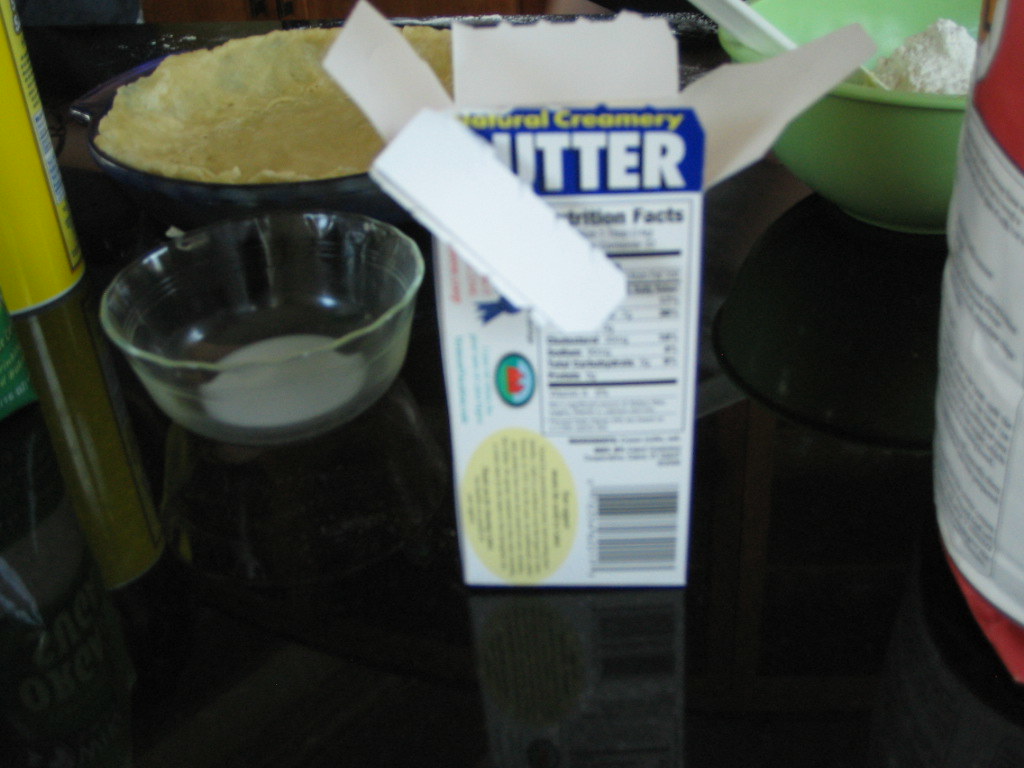This photograph captures an intimate and detailed scene of someone in the process of preparing a pie on a sleek, reflective black tabletop. Positioned at the center of the image is an opened container of butter, with its contents already removed. The back of the butter container faces the camera, revealing the partially visible label spelling out "UTTER" on a blue background, with the words "Natural Creamery" in bold yellow letters prominently displayed above. Beneath this, a Nutrition Facts label and a UPC code, along with various other text and graphics, can be seen on the left side of the container.

To the left of the butter container sits a clear glass bowl containing a white substance, likely pie dough or another baking ingredient, viewed from above. Behind this bowl is a pie plate already filled with a neatly pressed pie crust, ready for the next steps in the pie-making process.

On the right side of the butter container, a light green bowl filled with flour is visible, featuring a white spatula resting inside. Further to the right, a package of flour is partially visible, characterized by its distinctive red coloration at the top, middle, and bottom of the packaging. This composition, rich in detail, paints a vivid picture of a baking endeavor in progress, evoking the textures and colors of the culinary setting.